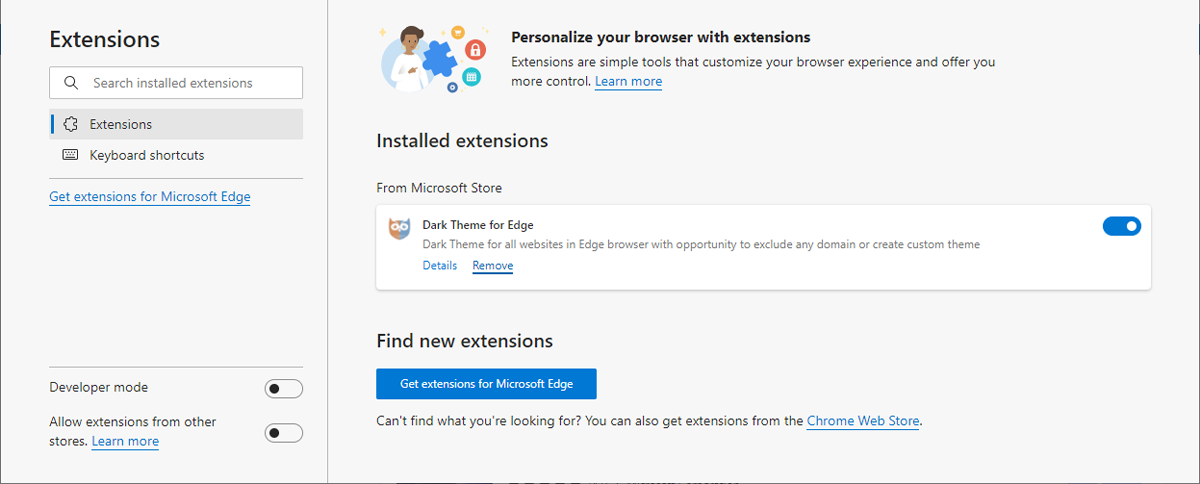This screenshot showcases a menu interface from an app or website, featuring a light gray background. On the left side, a vertical rectangle is headed by the label "Extensions." Below this heading, a white search field with a magnifying glass icon is placed, inviting users to "Search installed extensions." The next item is a highlighted "Extensions" option, followed by "Keyboard shortcuts." Further down, a clickable link titled "Get extensions for Microsoft Edge" is displayed. Below it, the label "Developer mode" appears with a switch to toggle it on or off. Additionally, there is an option labeled "Allow extensions from other stores" with a corresponding click area.

Adjacent to this vertical panel, on the right, the space transitions into a horizontal gray rectangle. Here, at the top, a header prompts users to "Personalize your browser with extensions." Farther to the right, an icon illustrates a cartoon of a Black woman holding a blue puzzle piece, accompanied by a description stating, "Extensions are simple tools that customize your browser experience."